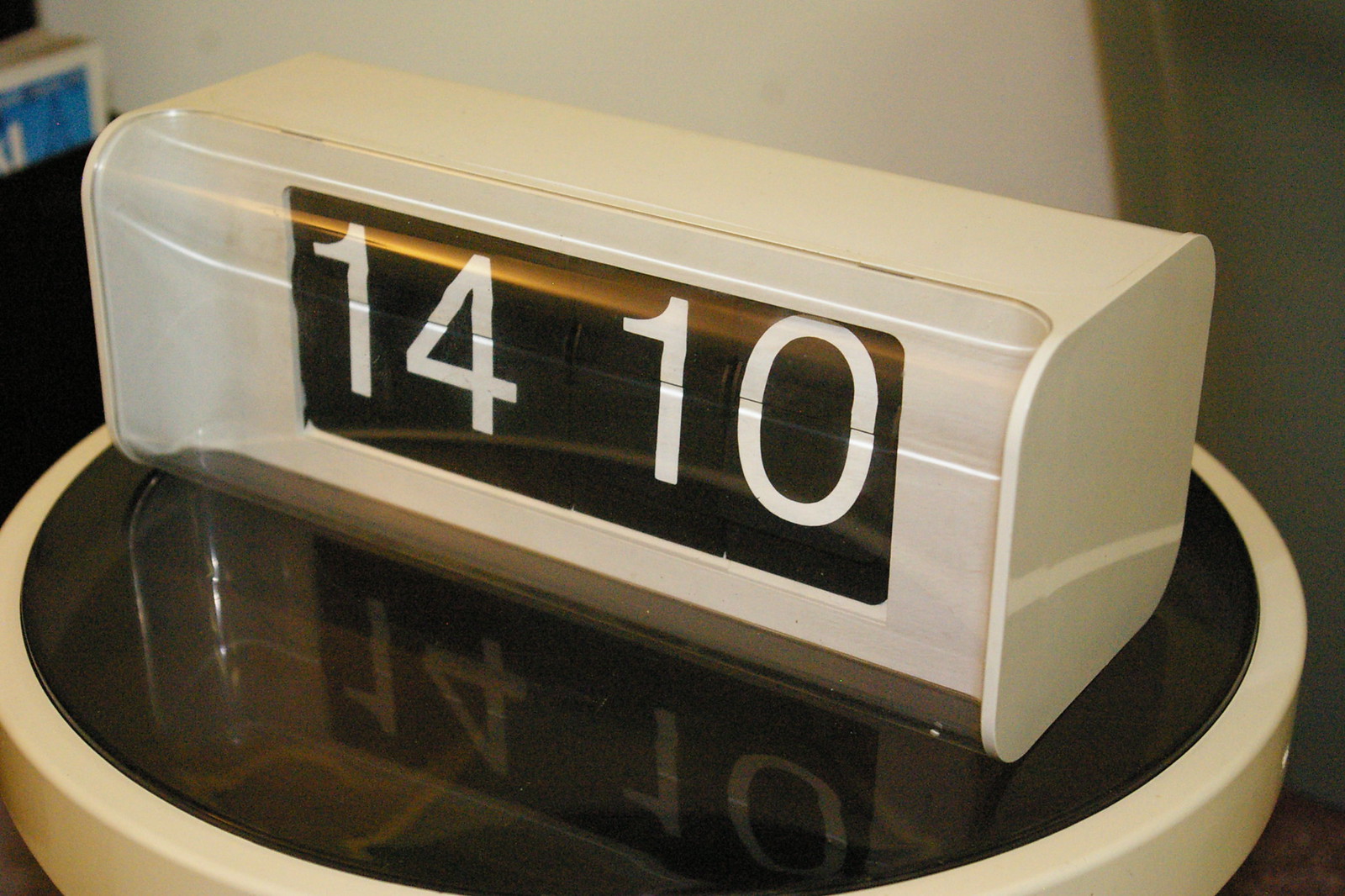The image depicts a digital white clock displaying the time "1410" in white numbers on a black face. This clock, which is rectangular with rounded edges, is positioned on a small, round table with a black reflective glass top and a white edging. The table itself appears to be part of a room with a white wall and possibly a doorway or entrance visible to the left side of the image. A bluish object, perhaps a book, is seen sticking out from the side of a table or chair in the background.